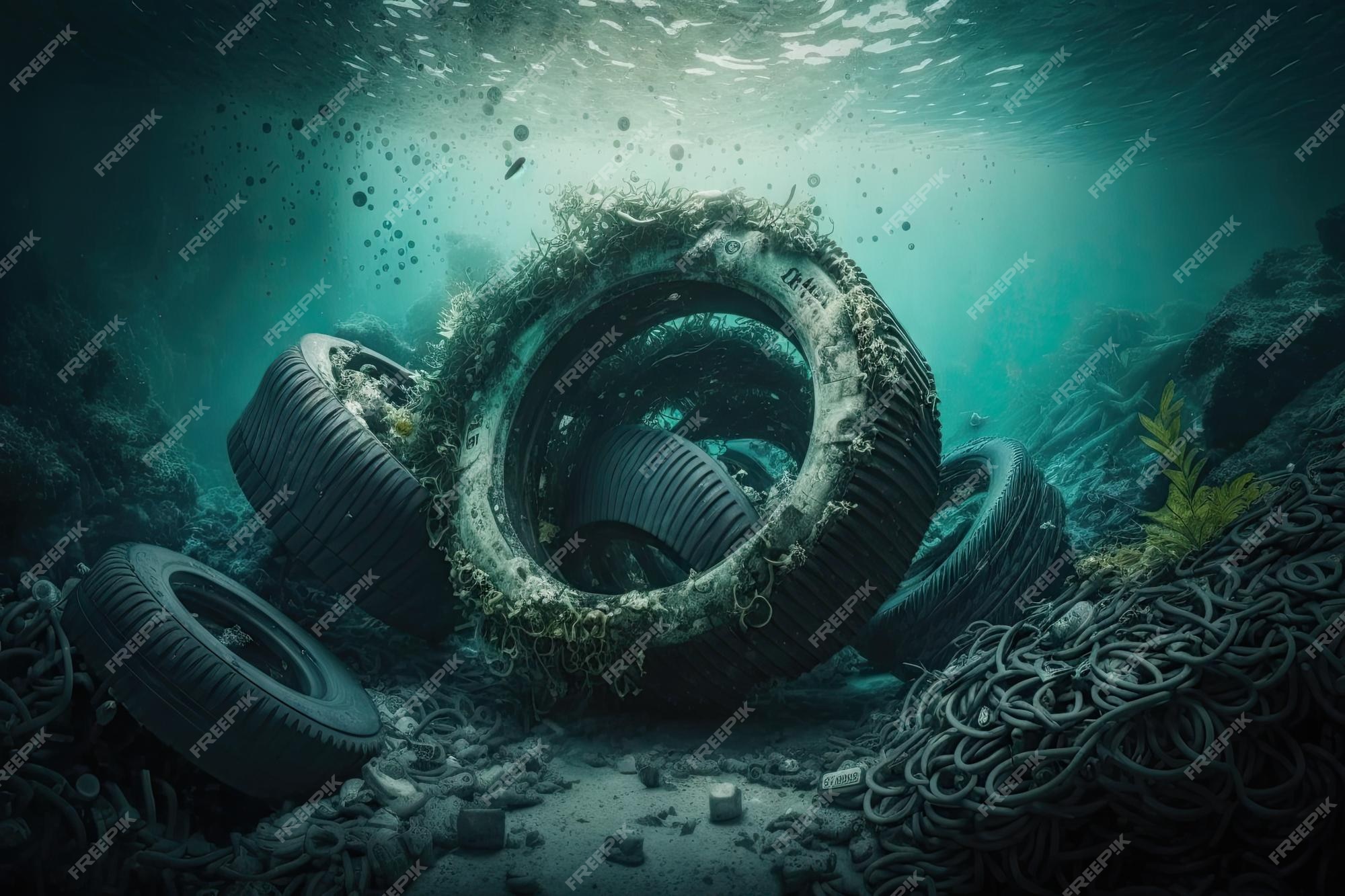This is a detailed, computer-generated underwater image depicting pollution at the bottom of a body of water. The water is an aqua blue color with sunlight filtering through, illuminating the scene beneath. Various old tires, around five or six, are scattered across the bottom. The central tire is heavily covered with moss and seaweed, indicating it has been submerged for a long time, while the others are relatively cleaner. To the right of this tire, there are tangled ropes or hoses, contributing to the overall sense of discarded waste. The water appears clear, but with no visible sea life, highlighting the bleak scene of pollution. Additionally, oil seems to be leaking from the central tire, creating floating oil bubbles that are rising towards the water's surface, further indicating contamination. The image features a watermark from "Freepik" that appears diagonally across the background. This composed image underscores the environmental impact of human littering, portraying an underwater junkyard of tires, ropes, and other debris.